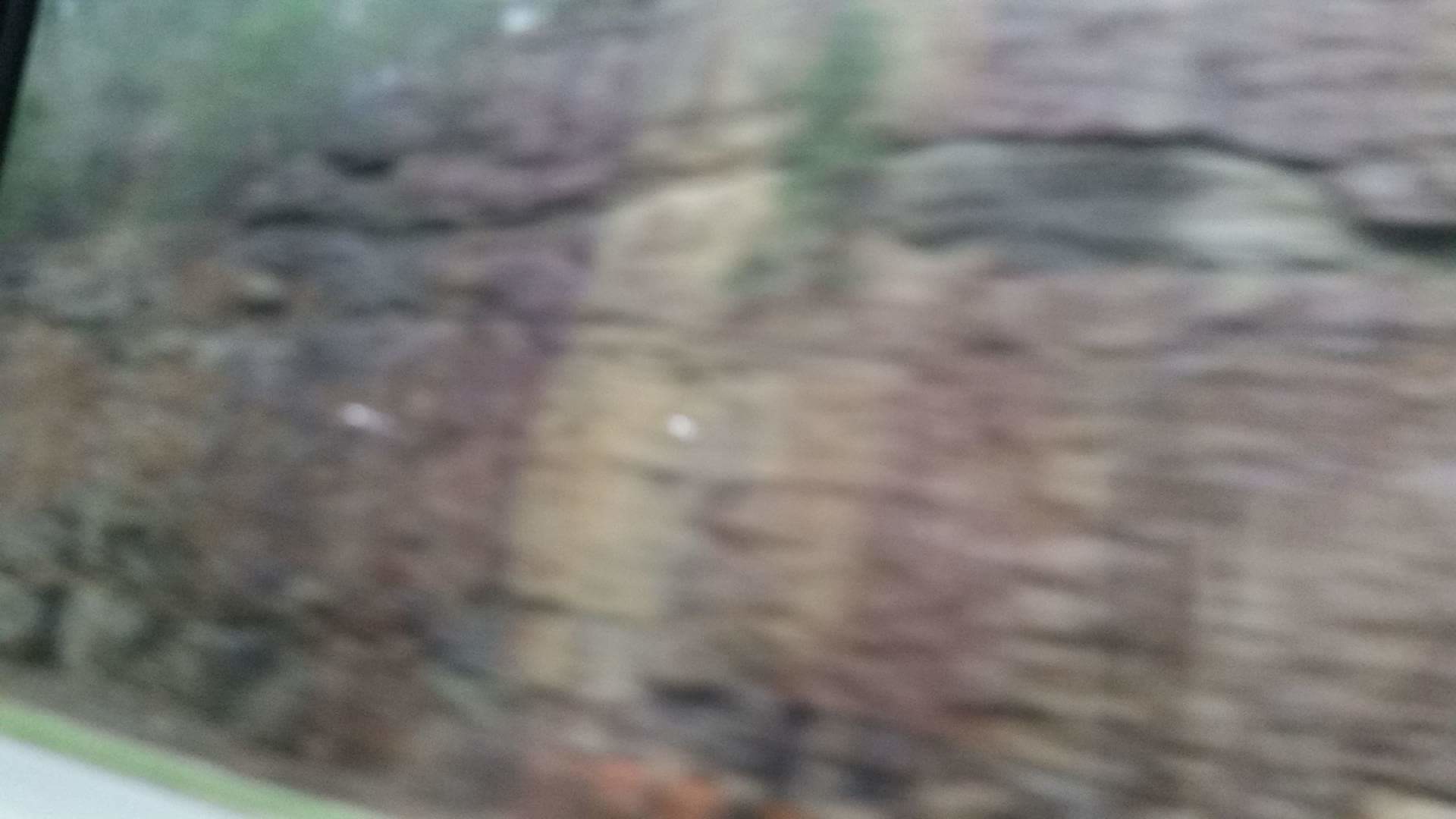This is a very blurry and indistinct color photograph that captures a close-up view of a massive rock-like structure, possibly an agate or slate formation, juxtaposed against a cliff or smoother mountainside. The image features a series of vertical strata composed of various colors, including shades of green, dark red, light tan, and purple, with darker and lighter bands slightly tilted to the right. The texture appears rough, and the strata's sequence extends from the bottom to the top of the photo. A noteworthy detail is the green strip in the lower left-hand corner, which might denote a strip of lawn, followed by a light gray area that could signify a road, potentially suggesting this rock formation was exposed during road construction through the mountain. The upper third of the image includes a larger band with streaks of white, gray, green, light yellow beige, and darker gray. Additionally, a slight black background appears in the top left corner, adding to the chaotic but fascinating blend of colors and textures.